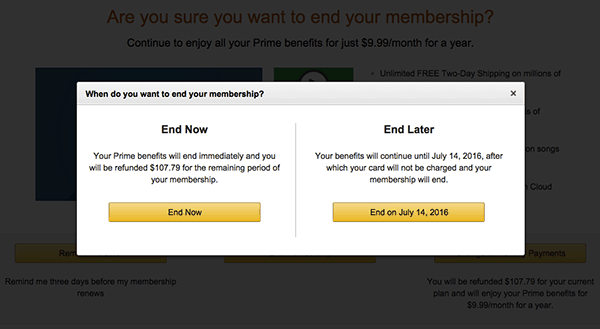The screenshot displays a computer screen with a pop-up prompt obstructing most of the background. The gray-tinted background hints at an interface where a user is attempting to cancel a membership. Despite the overlay, readable text suggests the user is canceling a Prime membership, with a red-tinted heading asking, "Are you sure you want to end your membership?" Additionally, text further down encourages continuing for $9.99 per month for a year, though much of it is obscured.

Dominating the screen, the pop-up window is a large white rectangle with a gray banner at the top featuring an 'X' for closing the prompt. The banner restates the concern with, "When do you want to end your membership?" Below, two options are visible: 

- On the left, a selection labeled "End Now" with a yellow button allows immediate termination of membership. The prompt clarifies that Prime benefits will end instantly and the user will receive a refund of $107.79 for the remaining period.

- On the right, a selection labeled "End Later" with a gold button gives the user the option to retain membership benefits until July 14, 2016, after which the membership will terminate, and no further charges will be applied.

Each option is clearly laid out with corresponding buttons — "End Now" on a yellow rectangle and "End on July 14, 2016" on a gold banner — providing a straightforward choice for the user.